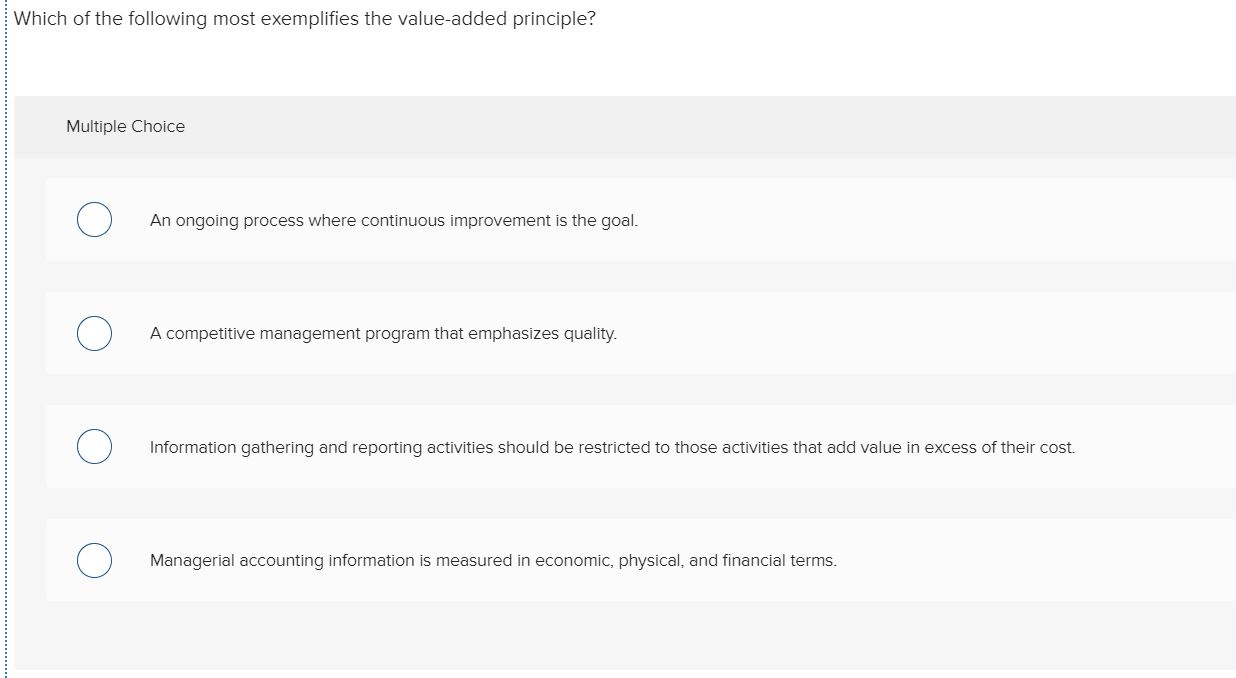Sure, here is a descriptive and detailed caption for the image:

---

In this digital image, a question is posed at the top in bold black font, asking, "Which of the following most exemplifies the value added principle?". Below the question, several multiple-choice options are presented within individual bubbles. The first bubble states, "An ongoing process where continuous improvement is the goal." The second option reads, "A competitive management program that emphasizes quality." The third choice articulates, "Information gathering and reporting activities should be restricted to those activities that add value in excess of their costs." Finally, the last option says, "Managerial accounting information is measured in economic, physical, and financial terms." The image aims to test the viewer's understanding of the value added principle in the context of managerial accounting and business processes.

---